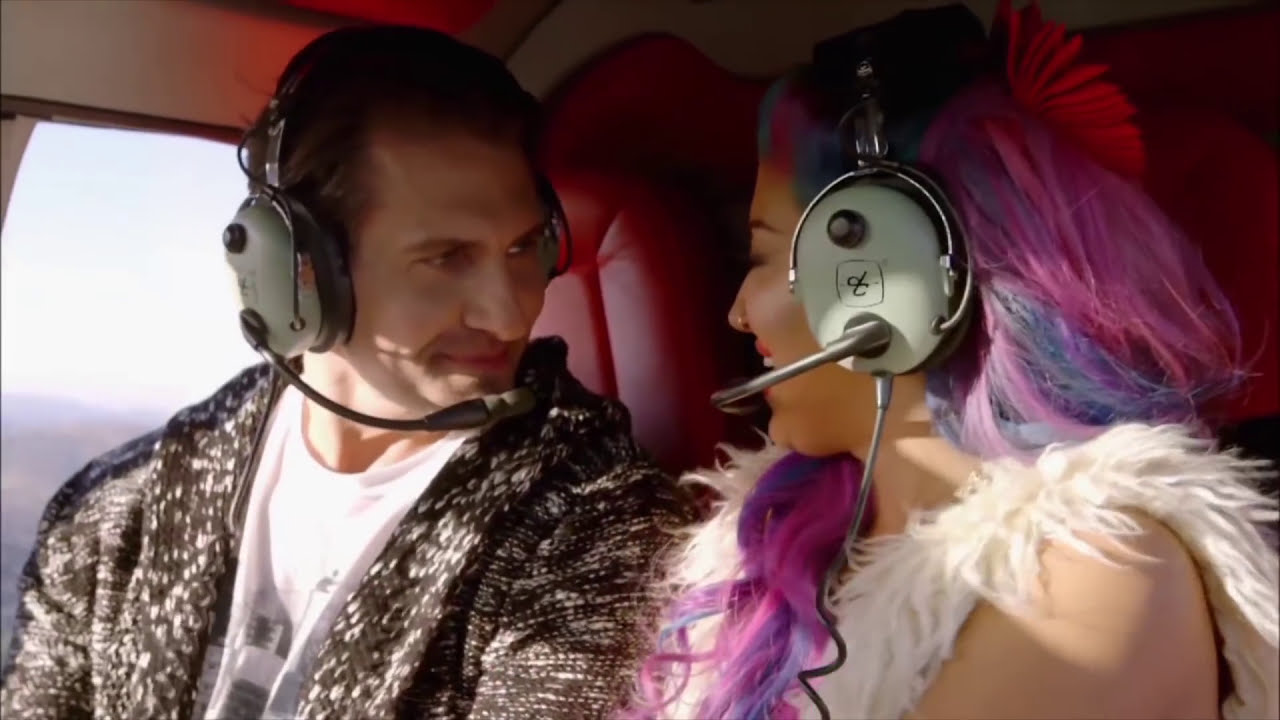The photograph captures an intimate moment between a man and a woman seated in the back of a helicopter. Both are dressed in headsets featuring thick, gray earpieces with attached black microphones and a stylized cursive "T" symbol in black. The man, positioned on the left, has short, dark hair and is clean-shaven. He is wearing a white t-shirt beneath a black and white light jacket and is giving a closed-mouth smile, intently gazing at the woman. The woman, seated on the right, is smiling widely back at him. She has vibrant pink and purple hair adorned with a red flower, tanned skin, and a nose ring. She is dressed in a fuzzy white, sleeveless top that resembles rabbit hair. They are seated on red leather seats with matching headrests, and through the window behind them, a hazy white sky and indistinct ground can be seen. The atmosphere is one of tender connection as they look at each other, surrounded by the bold red interior of the helicopter.